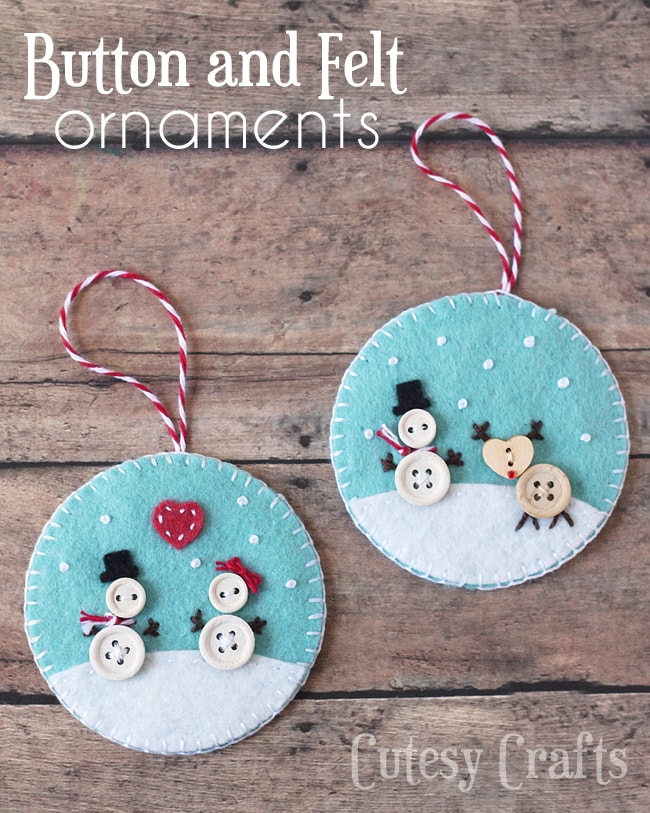This color photograph, in portrait orientation, showcases two handmade felt ornaments with buttons set against a weathered, light brown wooden platform with black marks. At the top left of the image, white text reads "Button and Felt Ornaments," while in the bottom right corner, light white text spells "Cutie Crafts." The ornaments are designed in blue and white felt, featuring intricate stitching along the edges. Both are circular and depict wintry scenes.

The ornament on the left hangs from a red and white knot and features a snowman crafted from two white buttons, with the smaller button on top. The snowman wears a black top hat and a red scarf, and a red heart embellishes the scene. The ornament on the right displays a similarly styled background with a white felt hill and an aqua sky dotted with small white buttons. This ornament showcases a snowman couple, with a male snowman button on the left and a female snowman button on the right, alongside a reindeer figure with a heart-shaped button head. The detailed craftsmanship and the realistic, representational photographic style highlight the charming, festive nature of these decorations.